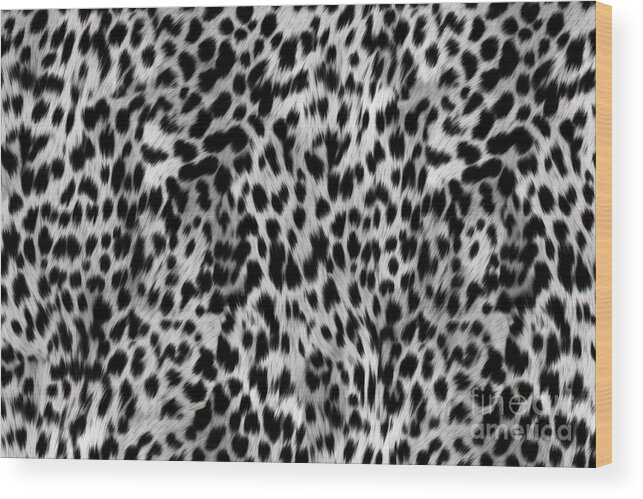The image is a detailed photograph of a rectangular board with a framed picture that covers its entirety. The picture showcases a white fur background adorned with numerous black spots, closely resembling a leopard skin pattern. The fur appears ruffled and textured, suggesting a three-dimensional, blanket-like quality, possibly indicating it is a throw or rug, though it's unclear if it is real or artificial. The frame itself has visible thickness, depicted as a brown, wood-like material on the right side of the board. In the lower right corner of the image, there is a semi-transparent watermark that reads "Fine Art America," blending into the intricate pattern of the depicted fur.